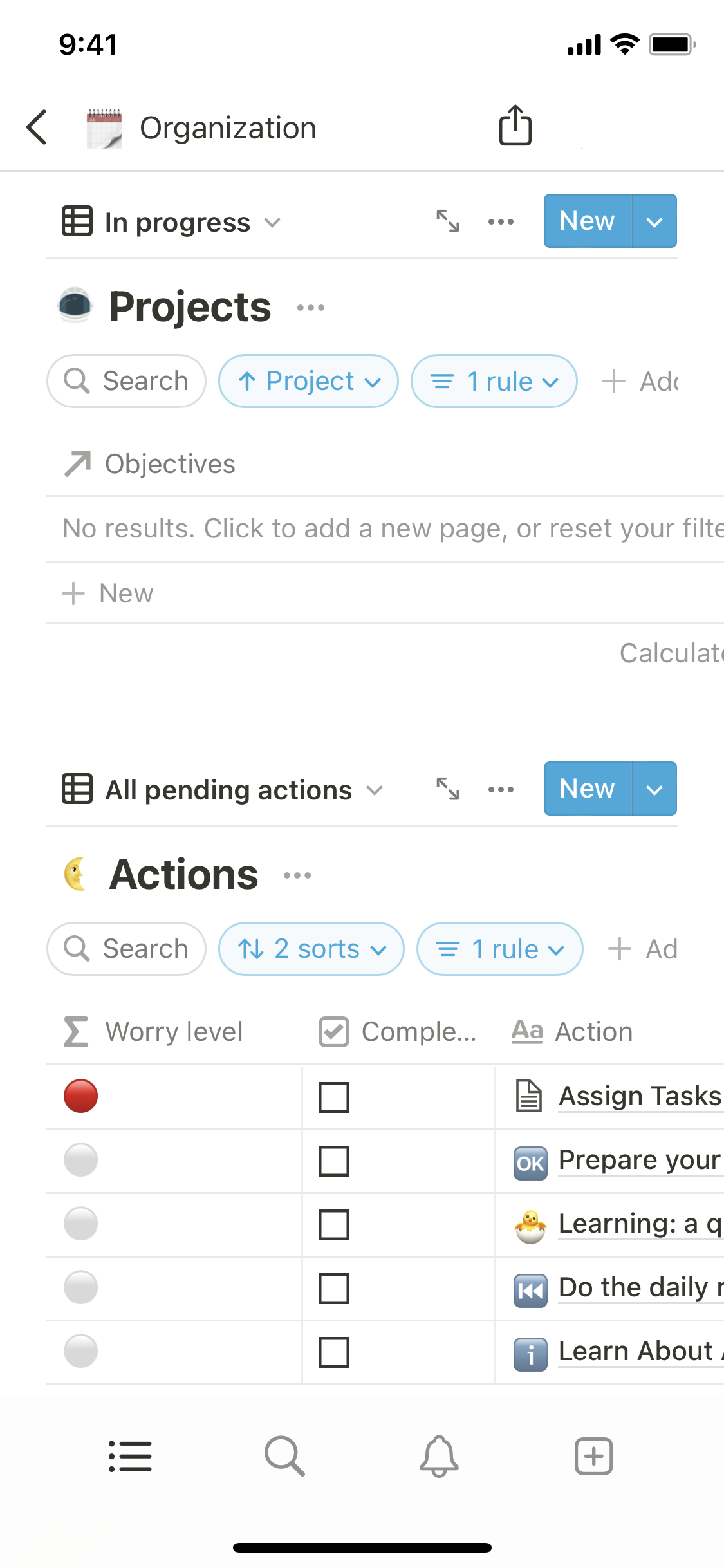**Website Category: Detailed View on Phone Screen**

The screenshot showcases a phone screen with a full battery, Wi-Fi enabled, and a signal strength displaying full bars. The time on the screen is 9:41, though it is unclear whether it is AM or PM. 

At the top of the screen, a calendar is visible with the heading "Organization: The Ability to Upload." Below this, the status "In Progress" is noted on the next line, accompanied by a dropdown menu for further options. On the same line, there is a blue box labeled "New," which also features a dropdown menu for additional functionalities.

Further down, a section labeled "Projects" appears, with an ellipsis icon to its right, indicating more options can be accessed by clicking. Beneath this, a search bar is present with the term "Project" specified, and a dropdown menu available for more filtering choices. Another heading, "One Rule," also includes a dropdown menu.

A partially obscured label reads "Plus AD," though the remainder of the text is not visible. Below this section, there is a category for "Objectives" showing no results, with prompts to either add a new page or reset the filter. 

Towards the bottom of the screen, the phrase "All Pending Actions" is displayed, paired with another "New" box that includes a dropdown menu. Lastly, the screen mentions "Actions," with features to search, sort twice by one rule, determine worry levels, and assign tasks.